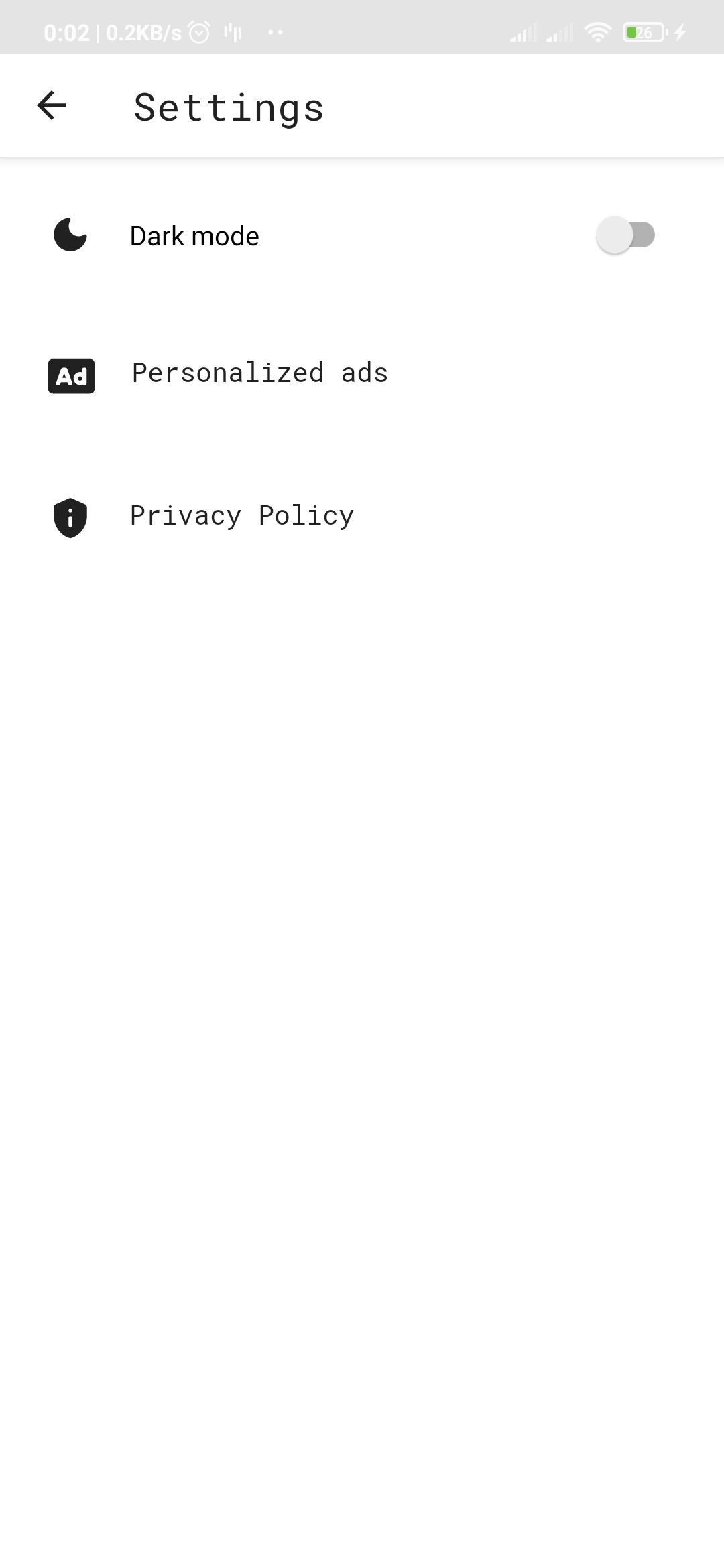The image is a screenshot captured from a smartphone's settings menu. The background is predominantly white, with a gray status bar at the top, displaying standard mobile information. The status bar includes the current time, shown as 00:02, and a data transfer rate of 0.2 KB/s. It also features an alarm clock icon, a series of signal bars indicating cellular network strength, and two white dots. On the far right of the status bar, there are more signal bars, a Wi-Fi connectivity icon, and a battery indicator showing 26% charge with a lightning bolt symbol, signifying that the device is currently charging.

Beneath the status bar, the settings section is displayed. An arrow pointing to the left is located at the top left, next to the word "Settings" in black text. Scrolling down, you'll find a toggle for Dark Mode, accompanied by a crescent moon icon, indicating that Dark Mode is currently turned off. Below it, options for "Personalized ads" and "Privacy policy" are visible, continuing the list of available settings.